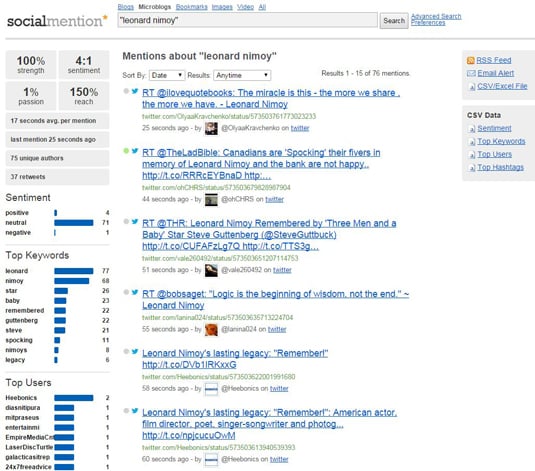The image displays a webpage from Social Mention, a social media analytics platform. In the upper left corner, the site's name, "Social Mention," is prominently featured. To the right, a search bar contains the phrase "Leonard Nimoy," with additional filtering options such as blogs, microblogs, bookmarks, images, video, and an option to view all mediums. The advanced search functionality is also available.

On the left side of the page, several gray information boxes provide detailed statistics: 
- 100% strength 
- 4 to 1 sentiment ratio 
- 1% passion 
- 150% reach 
- 16-second average per mention 
- Last mentioned 25 seconds ago 
- 75 unique authors 
- 37 tweets

Below these metrics, sentiment is broken down into positive, neutral, and negative categories. The section also highlights top keywords like "Leonard Nimoy" and "star," and phrases such as "baby remembered." Additionally, it lists top users, complete with their usernames.

The central area of the page displays various mentions of Leonard Nimoy, sortable by date and relevance. These mentions include Twitter posts from different users, each timestamped (e.g., 25 seconds ago, 40 seconds ago, 95 seconds ago), providing a real-time snapshot of social media activity related to the search phrase.

The page design is minimalist with a white background and straightforward text and search box layout, devoid of any elaborate designs. This clean interface facilitates easy access to the information and tools necessary for social media analysis.